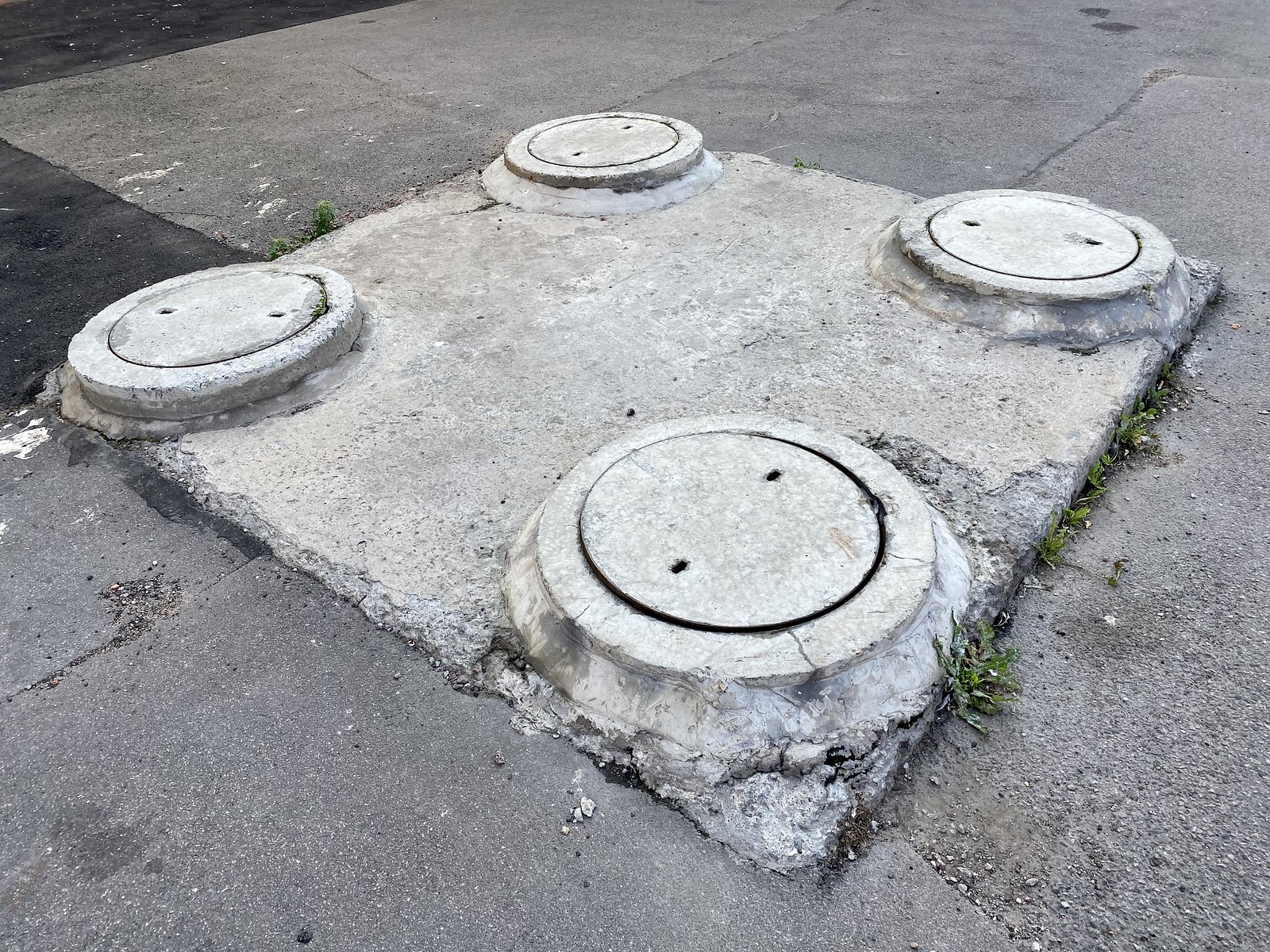The image showcases a section of urban landscape featuring a patchwork of various concrete and asphalt surfaces. Centrally located is a large, roughly square, semi-raised concrete slab, slightly elevated by about an inch, characterized by its chipped, poorly poured, and rough texture. This slab contrasts in color with its surroundings, appearing light gray or almost white against the darker gray concrete and black asphalt nearby. In each of the slab’s four corners, there are circular, flat-topped areas with manhole-type covers, complete with two slots presumably designed for removal tools or tongs, suggesting potential access points for utilities such as water mains, meters, or possibly sewer connections. The integration of newer, darker asphalt and older, gravelly concrete further highlights the patchwork nature of the area. Weeds and grass emerge from the cracks around the slab, indicating the structure's age and wear. Pebbles and debris around the edges of the concrete add to the sense of neglect and time-worn instability in this urban setting.